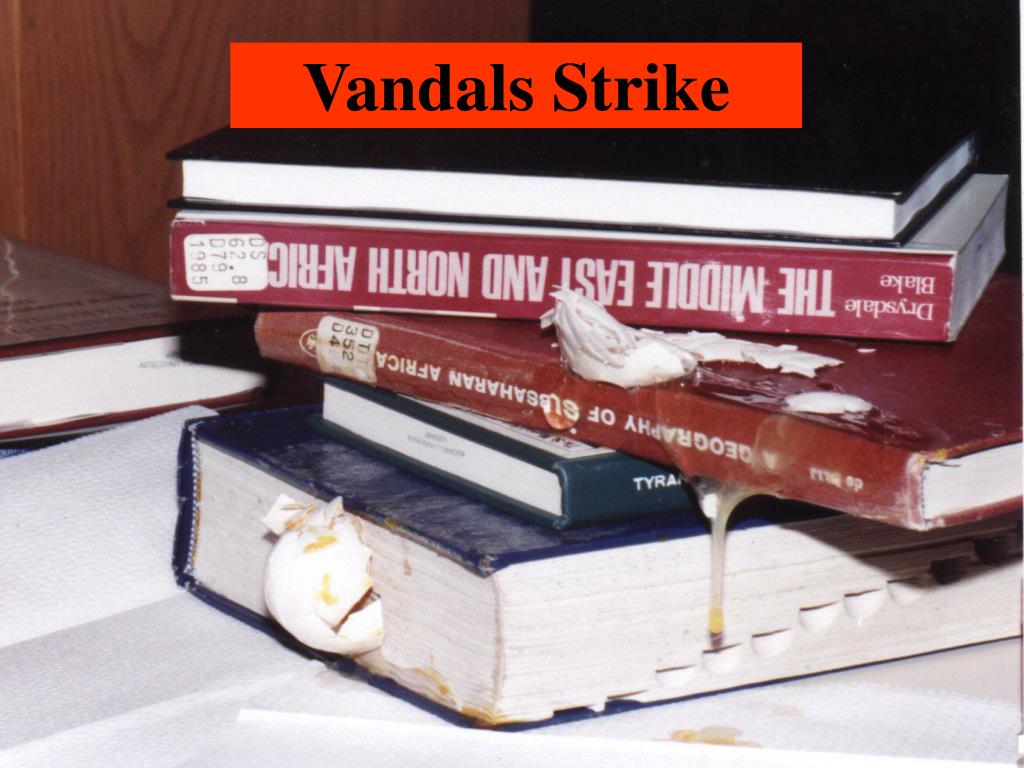In this image, a cluttered stack of books dominates the scene, with a wooden panel visible at the top, possibly from a wall or shelf. The left and right sides of the image are cast in shadow, appearing solid black. The books rest upon a white surface, likely papers on a desk or table. The stack consists of five books, arranged from bottom to top. The bottom book is thick, with a navy cover and white pages. Above it lies a smaller blue-green book, featuring the letters "T-Y-R-A" partially visible. Next, there is a thicker book with a burgundy cover, upside down, titled "A Geography of Caesarean Africa," identified by a black tag labeled DT35204. Above it is another red book with white cover edges, titled "The Middle East and North Africa" by Drisdale Blake, also upside down, tagged DS62.80791985. The topmost book in the stack is black with no visible title.

A mess of a cracked egg, complete with gooey contents and broken shell, drips down the middle of the stack, particularly onto the Geography book and the navy book below it. To the left, behind the stack, a brown book is visible. Finally, the image's title, "Vandals Strike," is prominently displayed in black letters against an orange rectangle at the top of the image. This chaotic scene suggests disturbance and mess, possibly in a library or school setting.